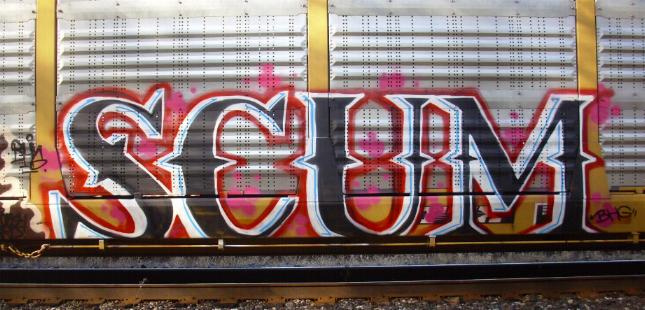This vibrant horizontal photo captures a detailed view of graffiti art on the side of a yellow and silver corrugated metal train car. Separating the panels of the train are yellow vertical metal beams, scattered with lines of small rivets. The graffiti features bold, black, 3D capital letters spelling "SCUM," prominently positioned across the corrugated surface. Each letter is meticulously outlined in white, followed by a red border, with touches of pink spray paint adding a subtle glow and sparse highlights around the lettering. Below the stopped train car, the dark brass-colored metal tracks are visible, supported by the gravel that forms the railroad bed, extending from left to right in the foreground.